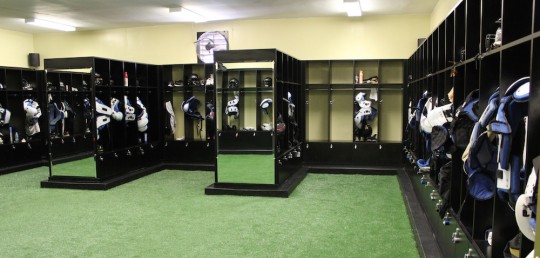This image depicts the interior of a vacant sports team locker room, possibly for a football or hockey team. The flooring is covered with green carpeting or artificial turf, and the room is illuminated by three long fluorescent lights mounted on a white ceiling. The walls are a pale yellow, adding to the stark ambiance of the space. Along the right side and extending to the far wall are rows of black locker cubbies, all open with various sports uniforms sticking out. These cubbies lack doors, exposing the contents within. At the far end of the room, two tall, vertical mirrors are positioned, reflecting more of the room’s elements. In addition, there is an island of lockers in the middle and smaller lockers at the front, maintaining the room's open and organized layout. The room is devoid of people, text, and animals, emphasizing its emptiness aside from the sports gear.